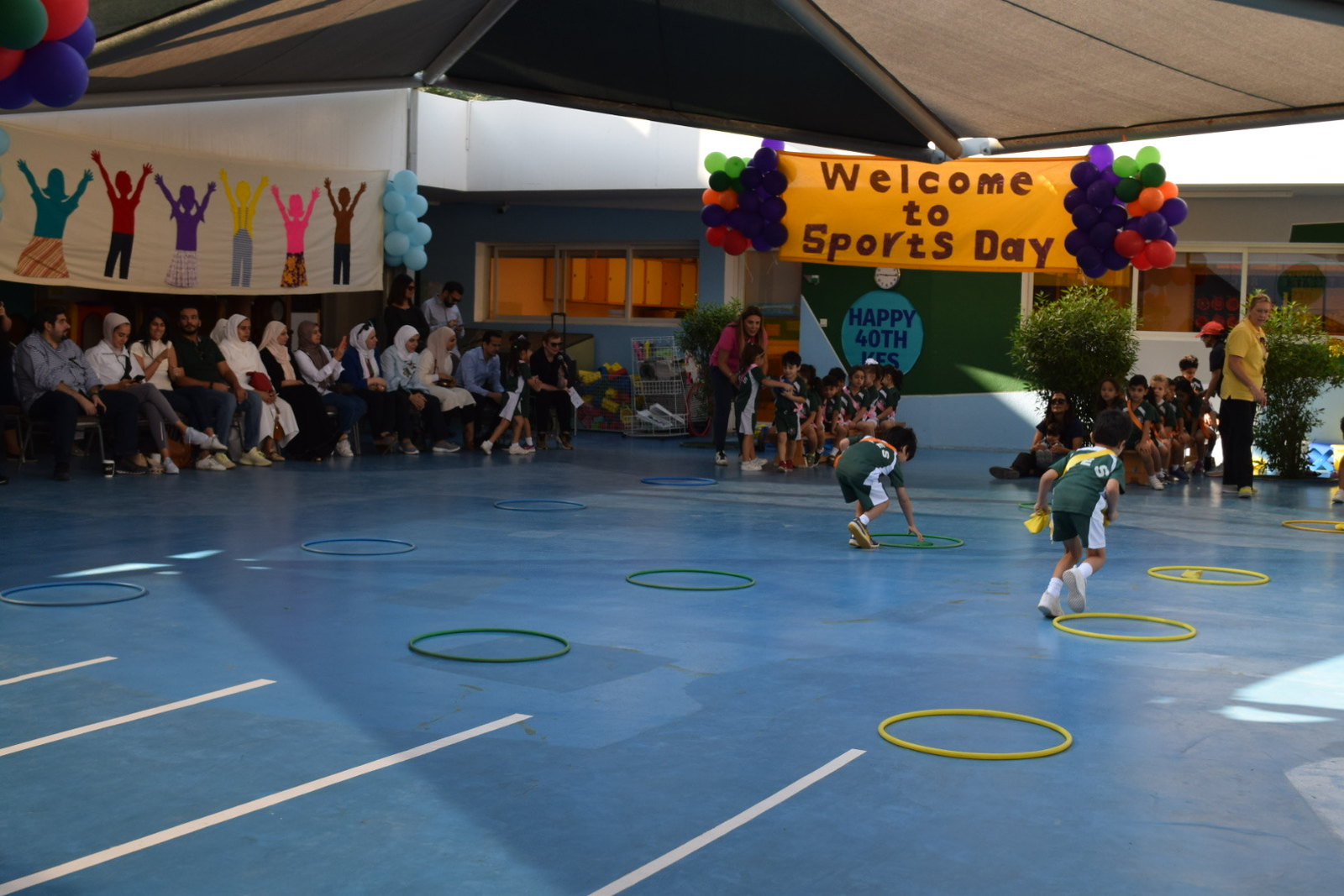The photograph depicts an indoor sports day event for children, held within a large building featuring a canopy-style green and white striped roof. The floor of the arena is a blue mat marked with white lines, suggesting a sports court. Arranged on the floor are rows of hula hoops in blue, green, and yellow, aligned from left to right. Two children wearing green uniforms are actively participating in a game; one is running along the yellow rings with his back to the camera, while the other is reaching into a green ring.

The room is filled with light, enhanced by the sun streaming in through large windows along the walls. A vibrant orange banner with red, purple, and green balloons hanging on either end reads "Welcome to Sports Day." Beneath this main banner, and framed by a small white wall, children dressed in various colors either sit or stand in anticipation of their turn. On another wall, there is a smaller banner adorned with multicolored graphics of jubilant children with raised hands, and more balloons.

Parents and teachers are seated in chairs along the edges of the court, attentively watching the children. Some teachers are also standing nearby, organizing and supervising the activities. The atmosphere is festive and dynamic, capturing the lively spirit of a school sports day celebration.